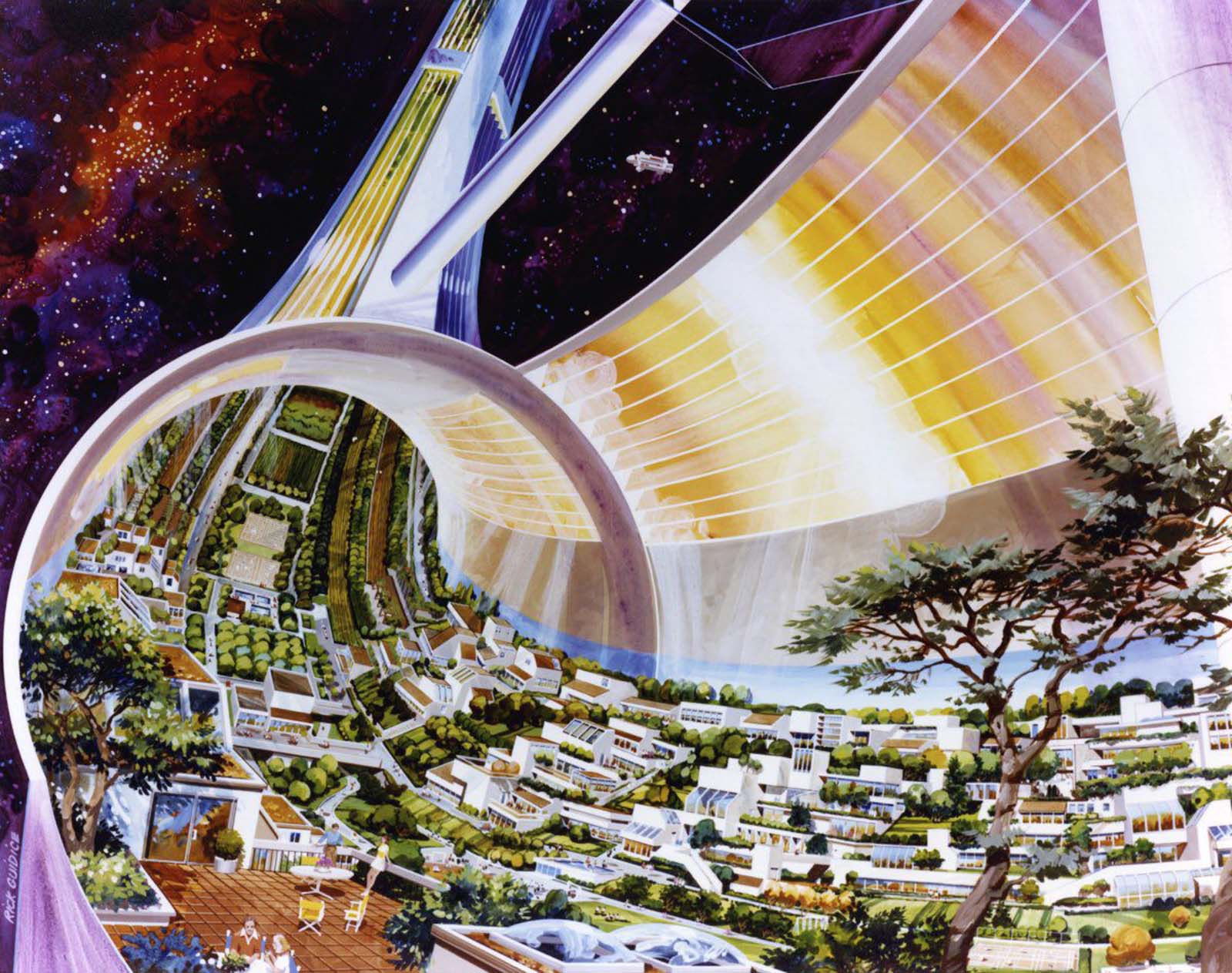This futuristic painting depicts a large, cylindrical tube-like structure seamlessly floating in space, possibly representing the outer ring of an advanced space station. The central top portion of the tube is connected to a support structure, suggesting its integration into a larger space habitat. The background vividly illustrates the cosmos with an array of nebulas, galaxies, and stars, showcasing vibrant hues of reds, blues, and purples against the blackness of space.

Inside the cylindrical structure, a meticulously detailed village unfolds. Agricultural plots and verdant gardens thrive alongside trees and numerous houses, which appear to ascend along the curve of the tube, defying traditional gravitational orientation. In the upper central part of the image, a small, silver spacecraft is visible in the distance, adding a dynamic element to the scene. This artwork beautifully captures the juxtaposition of natural greenery within a sophisticated spacefaring construct against a breathtaking cosmic backdrop.